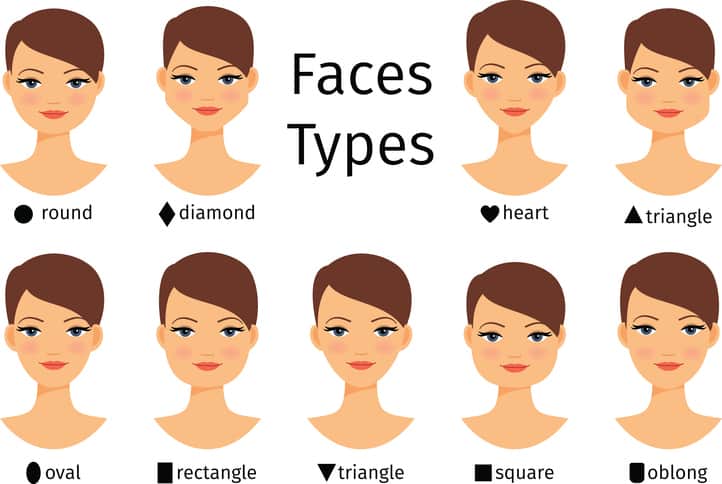This is a detailed poster illustration on a white background that showcases various types of human face shapes, organized into two rows. The top row features four face shapes depicted by cartoon women from left to right: round, diamond, heart, and triangle. The bottom row includes five face shapes: oval, rectangular, triangular, square, and oblong. Each face is portrayed by the same cartoon-style woman who is white-skinned, with blue eyes, pink lips, brown hair styled with bangs pushed to the side, and a slender neck. The poster positions all the women facing forward, and each face shape is accompanied by a small black icon illustrating the shape, along with the label of the face type. In the center of the graphic, separating the two rows, the wording "faces types" is displayed in black text.